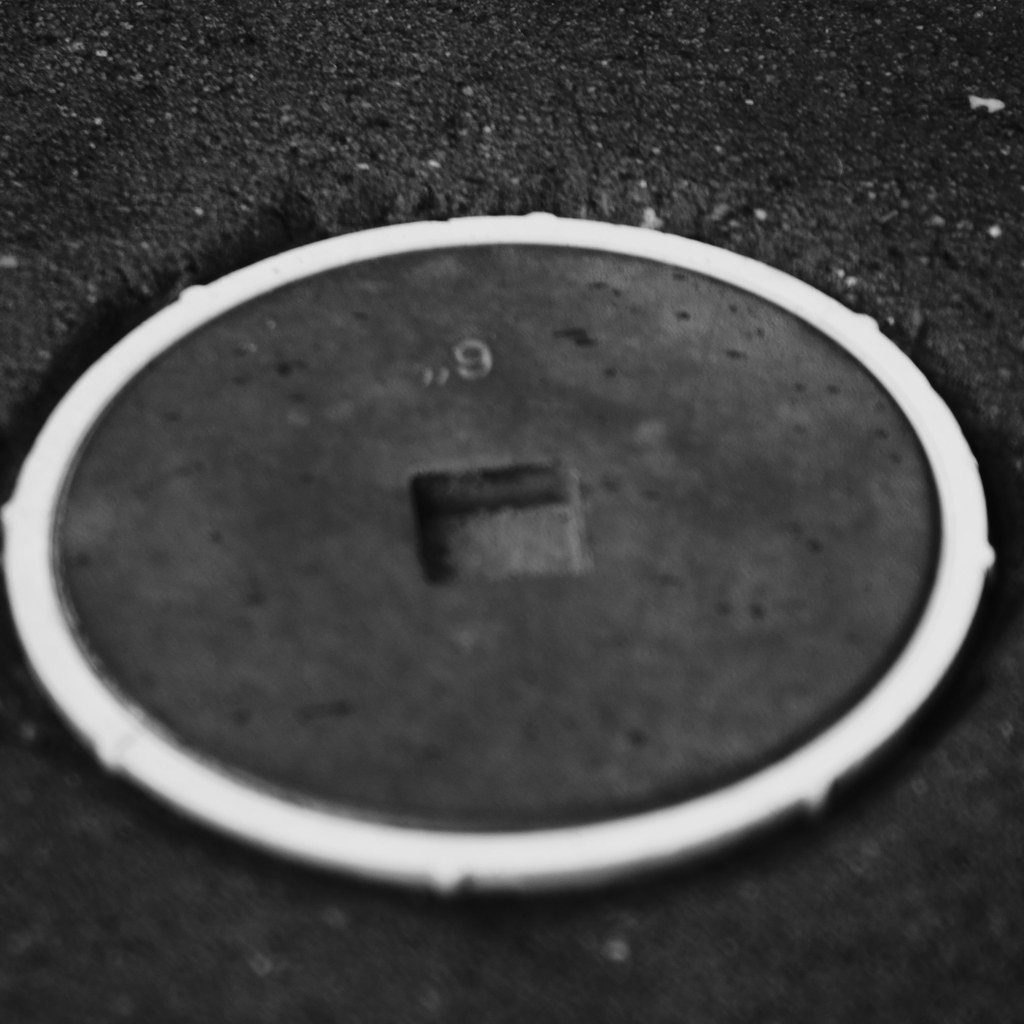A black and white photograph depicts a circular feature set into a cement or tarmac surface, resembling an industrial or road structure. The circle is outlined by a white rim with multiple raised notches, suggesting it is a cap or cover that can be unscrewed. Inside this white rim lies a flatter, smoother area of gray cement or concrete, contrasting with the rougher surrounding texture. At the center of the circle is a square indent, and above this indent is a marking that appears as the number six with two quotation marks when viewed in the photograph's orientation, but likely signifies six inches. The notches around the rim are positioned at intervals, specifically at the 12, 2, 3, 5, 6, 8, 9, and 11 o'clock positions. The entire scene is slightly out of focus, especially towards the bottom, giving it a surreal quality. The background texture resembles black tarmac with gray flecks, further implying the setting is a road or street.